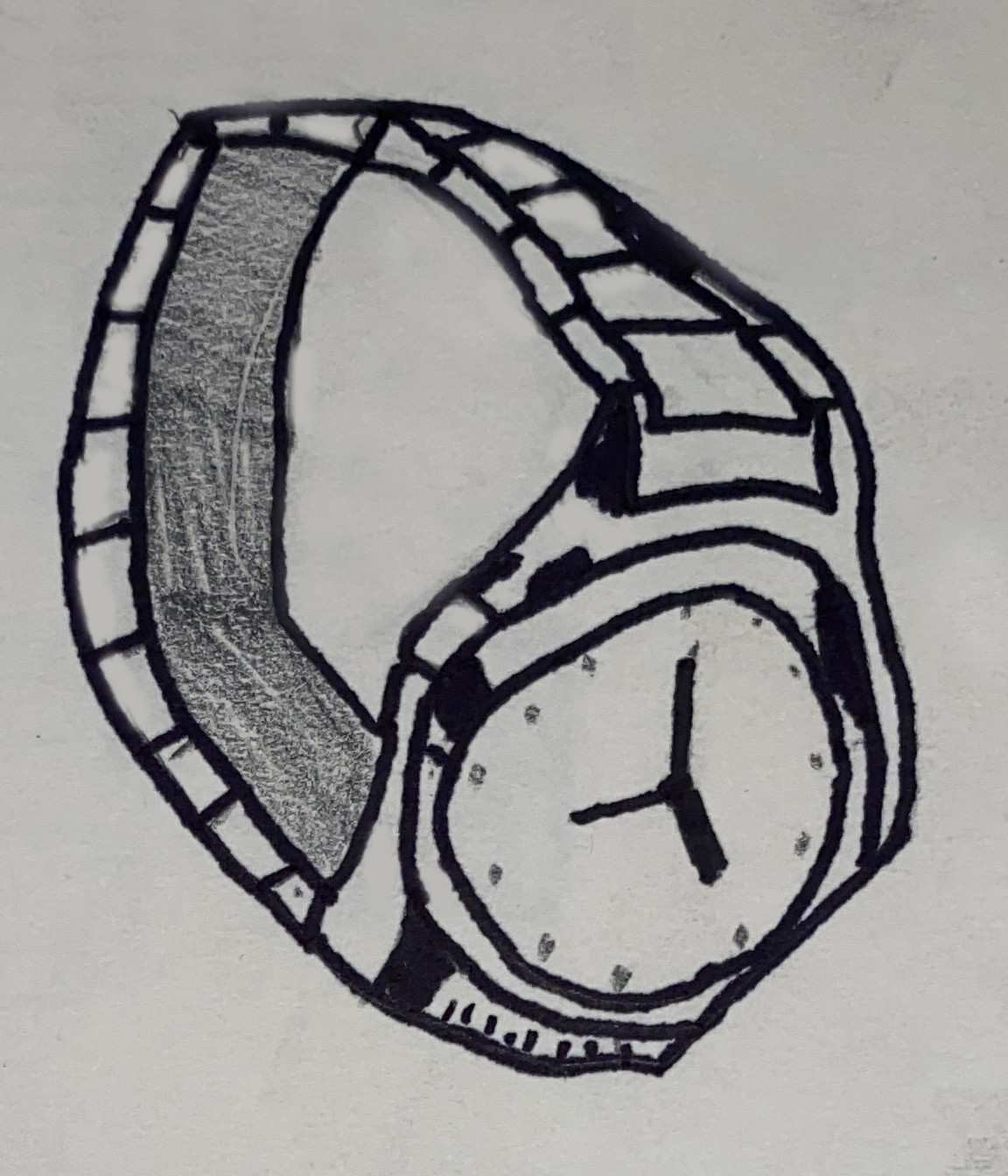This image is a highly detailed depiction of a wristwatch, crafted with a combination of crayon, color pencil, and marker on white paper. The watch is outlined with marker, and this outline reveals intricate details, including square-shaped links in the wristband. The face of the watch shows the time at approximately 5 o'clock, with thick, dark black hands for the minutes and hours, and a thin black second hand. The numbers on the watch face are represented by small dots, rather than numerals. The interior of the wristband is shaded with a gradient from light black to dark gray, offering depth and texture. The background paper shows a faint black brushed effect, possibly made by lightly skimming a crayon across it, enhancing the sense of shadow and depth. Subtle wrinkles and darker gray shadows further enrich the portrayal, making the watch stand out against its background.